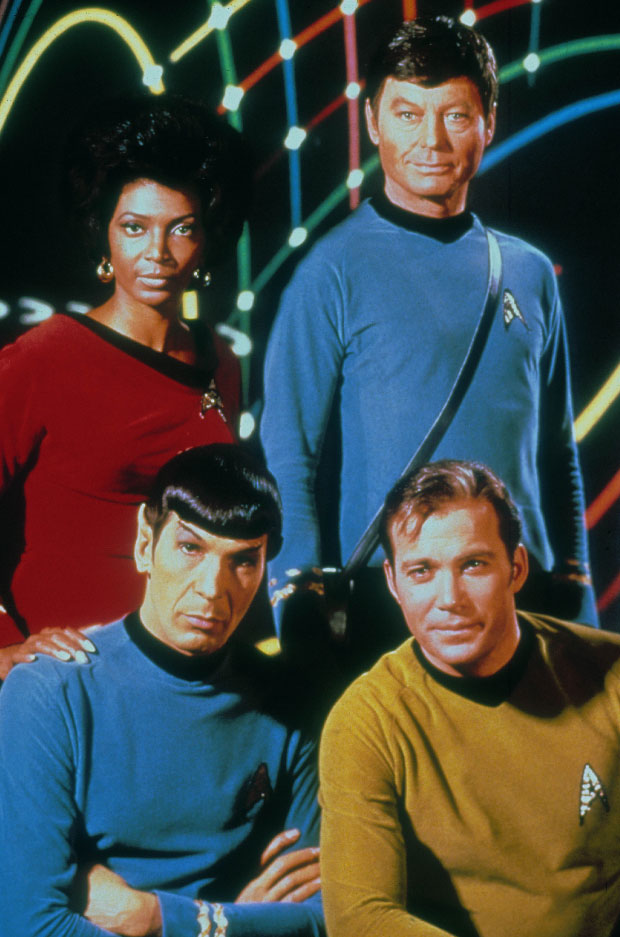This classic promotional image from Star Trek features four prominent characters set against a vibrant, 1960s-inspired background. Multicolored lines of pink, blue, orange, green, and yellow create a swirling pattern on a black backdrop, reminiscent of a latticework of LED lights. Positioned vertically, the image places Lieutenant Uhura in the upper left. An African-American woman, she sports a long-sleeve red uniform with a black collar, her hair either short or styled up, and gold hoop earrings. To her right is Dr. McCoy, a white man with short brown hair wearing a long-sleeve blue uniform, accented by a black medical strap across his chest, smiling warmly at the camera.

Seated in the lower left is Spock, displaying his characteristic serious expression. He has very short straight black hair with distinct bangs, pointed eyebrows, and is clad in a blue science officer uniform. To his right is Captain Kirk, easily identifiable by his light brown hair, blue eyes, and a gold command uniform. He wears a subtle, self-assured smile. This group, captured mid-pose against the kaleidoscopic yet dark background, perfectly embodies the essence of Star Trek's iconic series, bridging the bold attire of its characters with the vivid, futuristic style of its visual design.